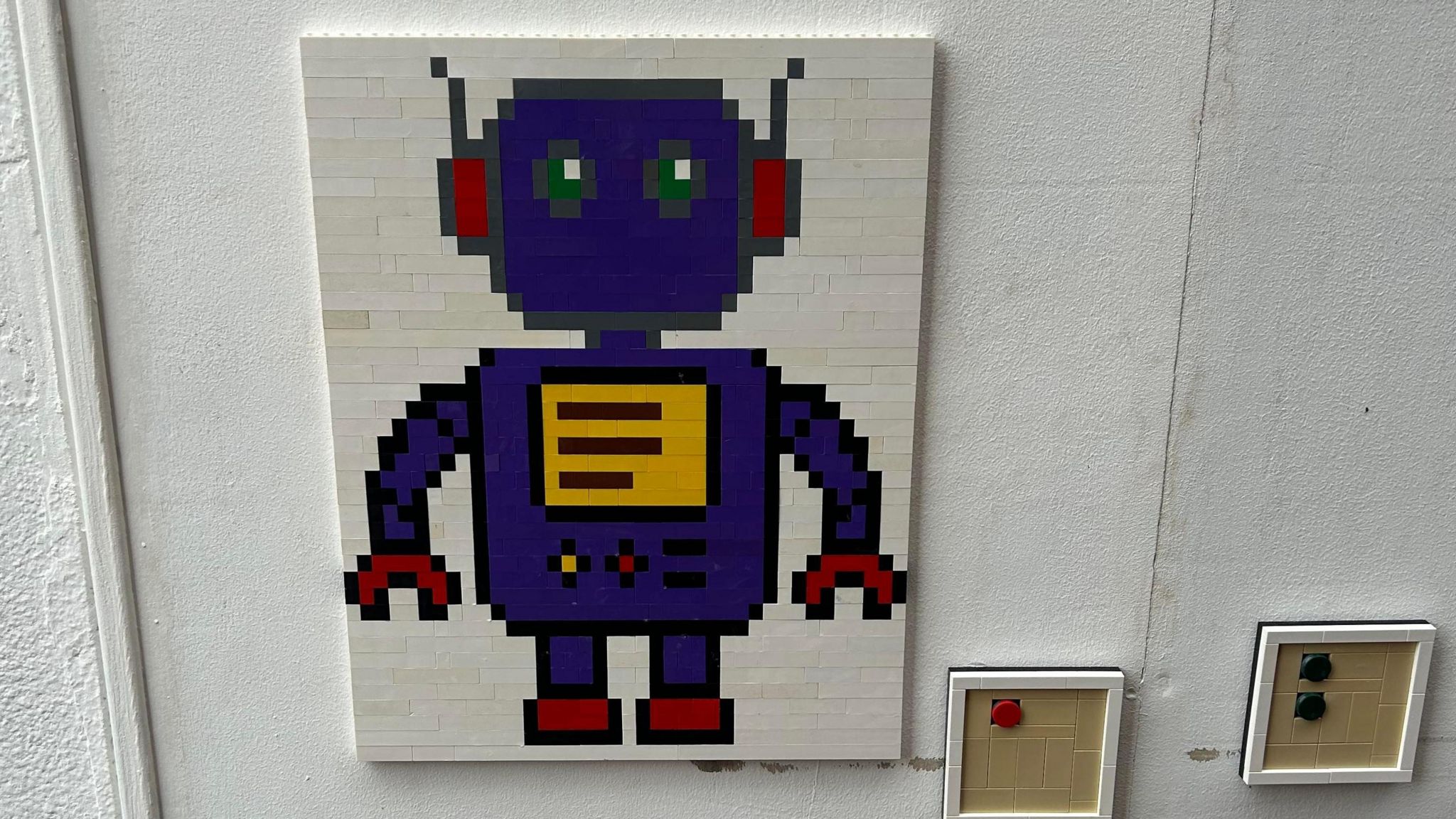The image depicts a detailed photograph of a piece of art constructed entirely out of Lego blocks, prominently featuring a robot against a white Lego-block background. The robot is predominantly blue with distinct red elements accentuating its hands, feet, and ears, which give it a colorful and playful appearance. Its head is square-shaped, adorned with gray plus-sign eyes that contain white centers. This minimalist robotic face is further characterized by what appear to be red headphone-like attachments near its ears.

The robot's chest showcases a notable control panel: a yellow-gold rectangular section with three black horizontal stripes and additional buttons, including a yellow button and a red button positioned lower on its torso. The control panel also features blue levers, illustrating the imagined control mechanisms of the robot.

In addition to the main robot figure, the piece also contains other Lego artworks to its right. These artworks similarly use a white Lego block outline and feature tan blocks within. One of these additional pieces has a single red button, while the other includes two green buttons, continuing the theme of interactive-looking controls.

This intricate Lego construction blends numerous vibrant colors such as red, yellow, blue, and emphasizes the detailed craftsmanship of using simple Lego blocks to create a sophisticated and engaging piece of art.